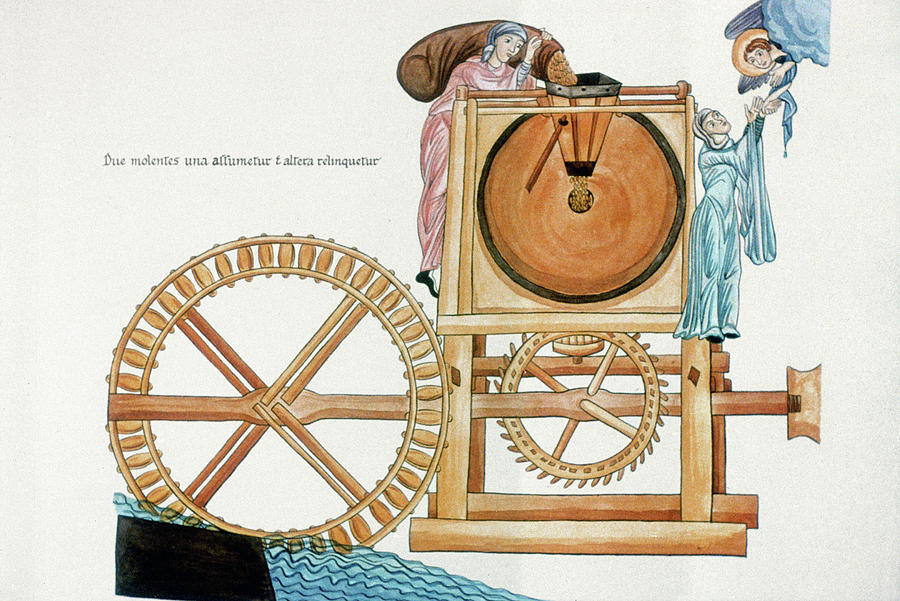The hand-drawn illustration depicts a traditional mill scene with two large wooden cogwheels powered by water. On the left side of the image, there is text in a foreign language which appears to be French, reading, "deux molins, une affumature, de l'altetta." A large water wheel is depicted semi-submerged in a flowing river, turning an axle that drives the cogwheels inside a tall, wooden mill structure. At the top of this structure, a woman in a blue dress is pouring grain into a hopper. Adjacent to this, on the right side, another woman in a blue dress reaches upward, where she is making contact with an angel descending from the heavens, depicted with a glowing halo. The background of the drawing features a pinkish off-white color, adding to the surreal and mystical nature of the scene. The image blends the practical elements of milling grain with expressions of celestial or divine intervention.